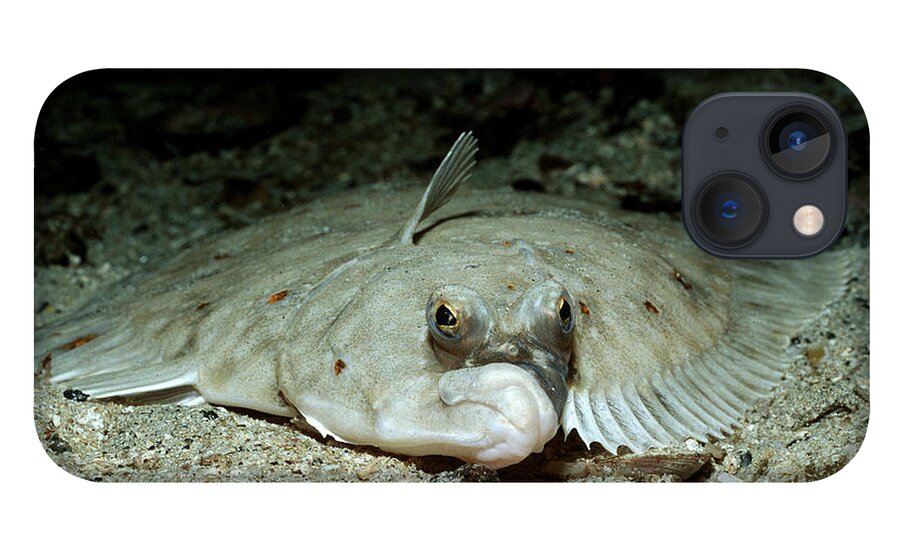This underwater photograph captures a flat sea creature resting on the ocean floor amidst a rocky, pebble-strewn background that appears cement-like. The sea creature resembles a stingray, with an expansive body, two prominent eyes, and distinct fins—one on top of its head and several gill-like fins on its sides. Its coloration is a mix of light gray, tan, and brownish gold spots that help it blend seamlessly with its surroundings. Above the creature, the image darkens toward the top left, giving a sense of depth to the underwater scene. In the top right corner, the design of a phone's camera module is visible, featuring two blue-lensed circles, a small black dot on the upper left, and a light tan dot on the bottom right. The phone camera design juxtaposes modern technology with the serene, natural habitat of the sea creature.